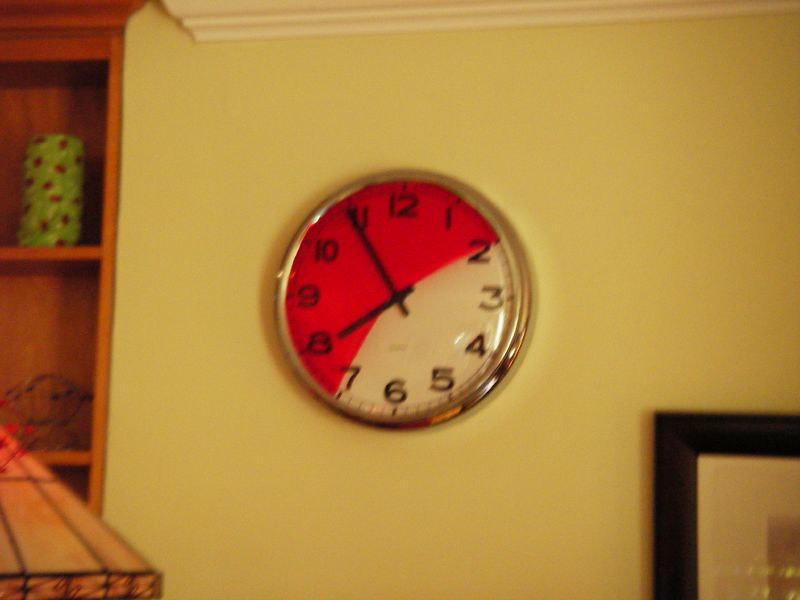In this low-resolution, blurry photograph, a circular wall clock featuring a silver border is prominently displayed in the center against a yellow wall. The clock's face is uniquely divided, with a red section spanning from the 7 to the 2 and a white section from the 2 to the 7. Its black numbers and hands read six minutes until eight o'clock. Above the clock, a white platform is visible. To the left, there is a brown, recessed bookshelf with at least two levels, where a vase is placed on the top shelf and a lampshade on a lower level. To the right of the clock, a part of a painting with a black frame and white border is partially visible, adding further detail to the setting.